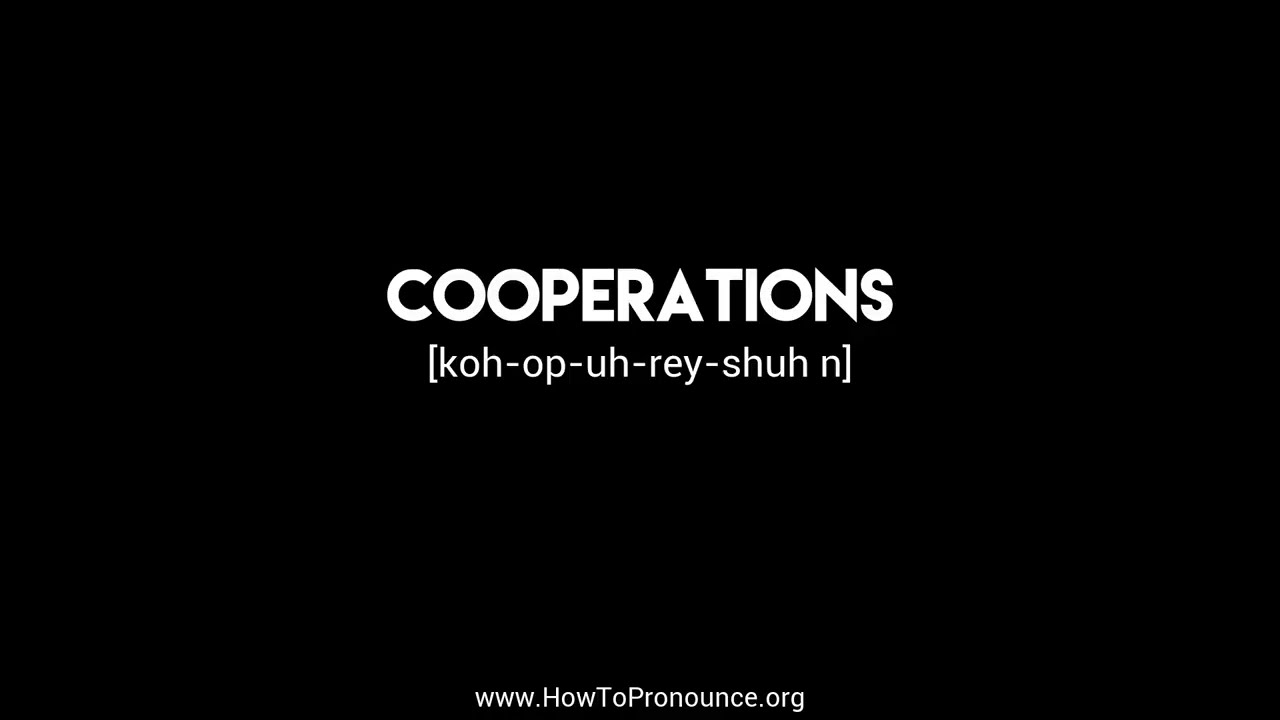The image features a solid black background with white text centered in the middle. The main text in all uppercase letters reads "COOPERATIONS," with a phonetic pronunciation written below as "K-O-H - O-P - U-H - R-E-Y - S-H-U-H space N." Notably, the pronunciation guide concludes with "space N" instead of "S." At the bottom of the image, in smaller white text, there is a web address: "www.howtopronounce.org," intended to assist users in learning the pronunciations of various words. The overall design is minimalistic, employing only black and white colors, and the layout is straightforward, with the word and its pronunciation centered and the web address at the bottom.